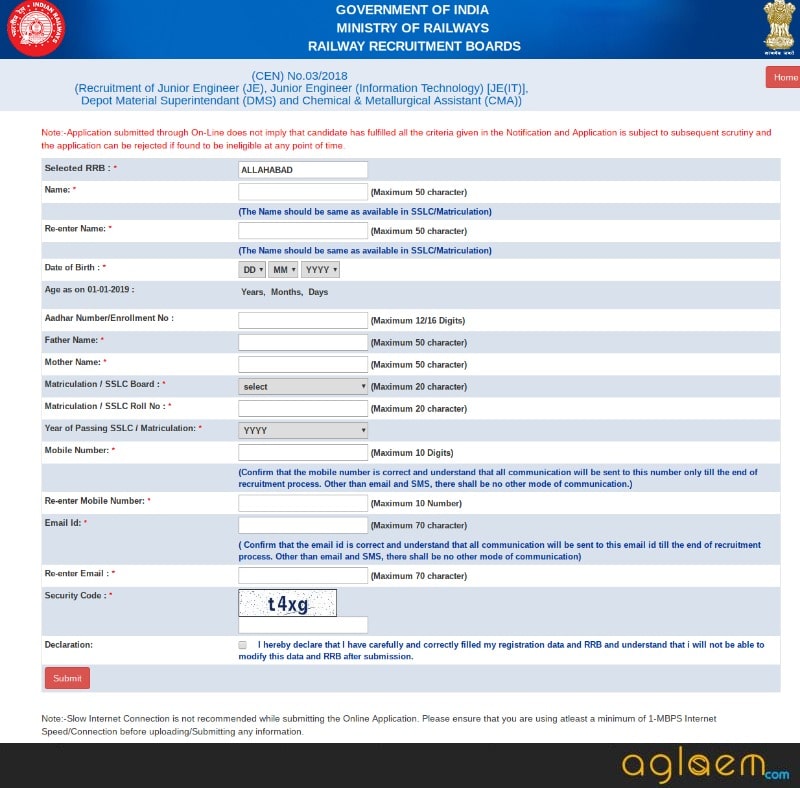Screenshot of the Government of India's Ministry of Railways - Railway Recruitment Board (RRB) job application page for the positions of Junior Engineer (Information Technology), Depot Material Superintendent, and Chemical and Metallurgical Assistant. The page header prominently displays the Ministry of Railways and Railway Recruitment Board insignia, followed by a clear disclaimer noting that the submission of an online application does not guarantee eligibility; applications are subject to further scrutiny and may be rejected if found ineligible at any stage.

Below, the form fields required to complete the job application are outlined:

1. **RRB Selection**:
   - Displayed location is "Allahabad" (assumed to be the municipality but is slightly blurred).

2. **Personal Information**:
   - **Name**: Two mandatory fields for name input, both allowing up to 50 characters, with a note to ensure consistency with SSLC/matriculation records.
   - **Date of Birth**: Input in DDMMYYYY format, with age as of 01/01/2019.
   - **Aadhaar Number / Enrollment Number**: Up to 12 or 16 digits.
   - **Father's Name**: Maximum 50 characters.
   - **Mother's Name**: Maximum 50 characters.
   - **Matriculation/SSLC Board**: Dropdown menu for selecting the appropriate board.
   - **Matriculation/SSLC Roll Number**: Up to 20 characters.
   - **Year of Passing**: Dropdown menu for selecting the year of passing.

3. **Contact Information**:
   - **Mobile Number**: Maximum 10 digits, with a confirmation field requiring re-entry.
   - Note: All communication will be conducted through this number and the provided email.
   - **Email ID**: Maximum 70 characters, with a confirmation field requiring re-entry.

4. **Security and Declaration**:
   - **Security Code**: Displayed as 'T4XG'.
   - **Declaration**: A mandatory affirmation that the information provided is accurate and understood to be unchangeable after submission.

5. **Submission Guidelines & Note**:
   - A reminder to ensure internet speeds of at least 1 Mbps for the successful submission of the application. 
   - A submit button is available to finalize the application.

At the bottom right corner of the screenshot, the website aglaem.com is noted.

This comprehensive form ensures all essential information is collected accurately and highlights the importance of fulfilling criteria and maintaining proper communication channels throughout the recruitment process.